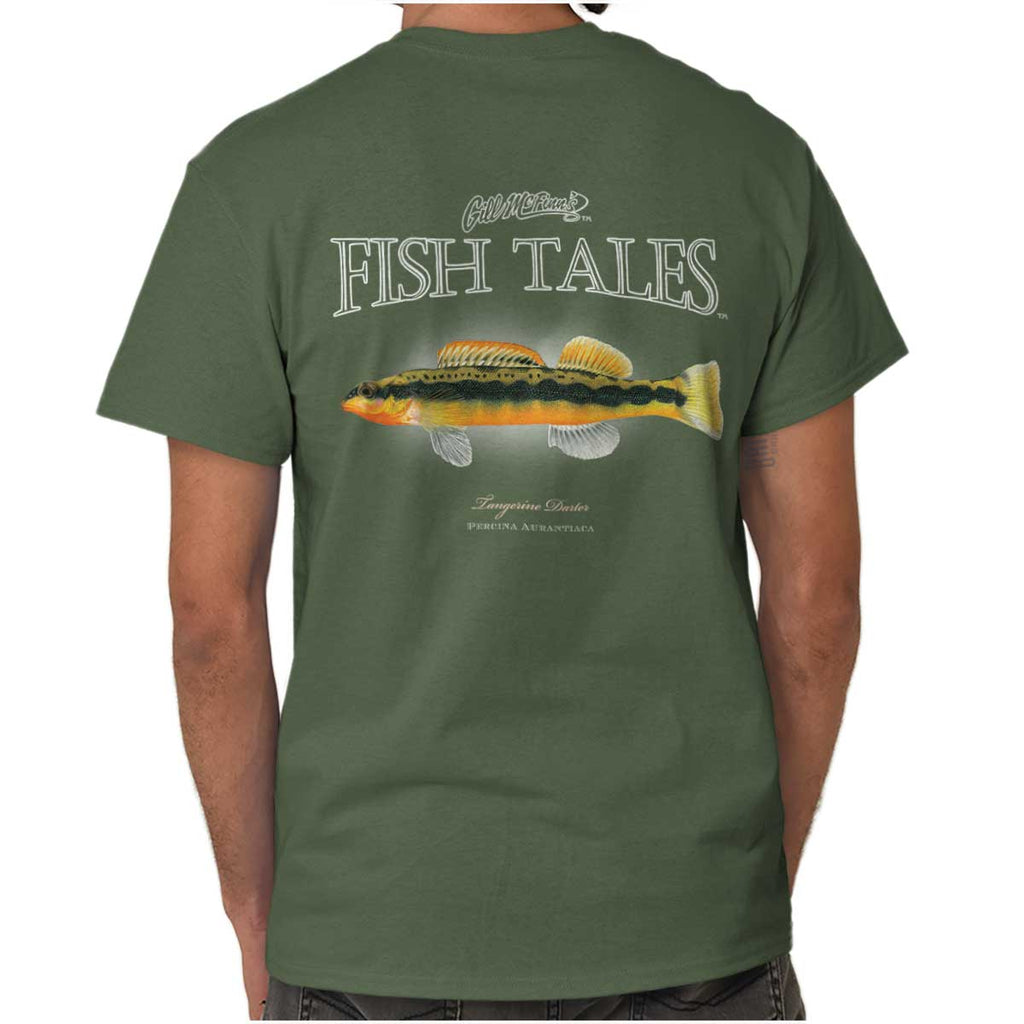The photograph captures a model from the back, showcasing an army green t-shirt, which appears slightly darker than olive. The model is a Caucasian man with lightly tanned skin, wearing faded black jeans and exposing a small, faded black line tattoo on the inside of his right bicep. The t-shirt, a crew neck, features a detailed design on its back. The top part of the shirt displays the words "Gil McFinn's Fishtails" in a combination of cursive and all capital letters. Below this text is a vibrant illustration of a long, skinny fish that is green and yellow with yellow-green fins. The fish faces left and has a notable, distinctive appearance, potentially indicating its species, although the small, stylized text beneath it, including "Priscina Orontiaca" and "Tangerine," is difficult to decipher. The model's elbows and the back of his neck are partially visible, contributing to the overall casual and detailed presentation of the shirt.